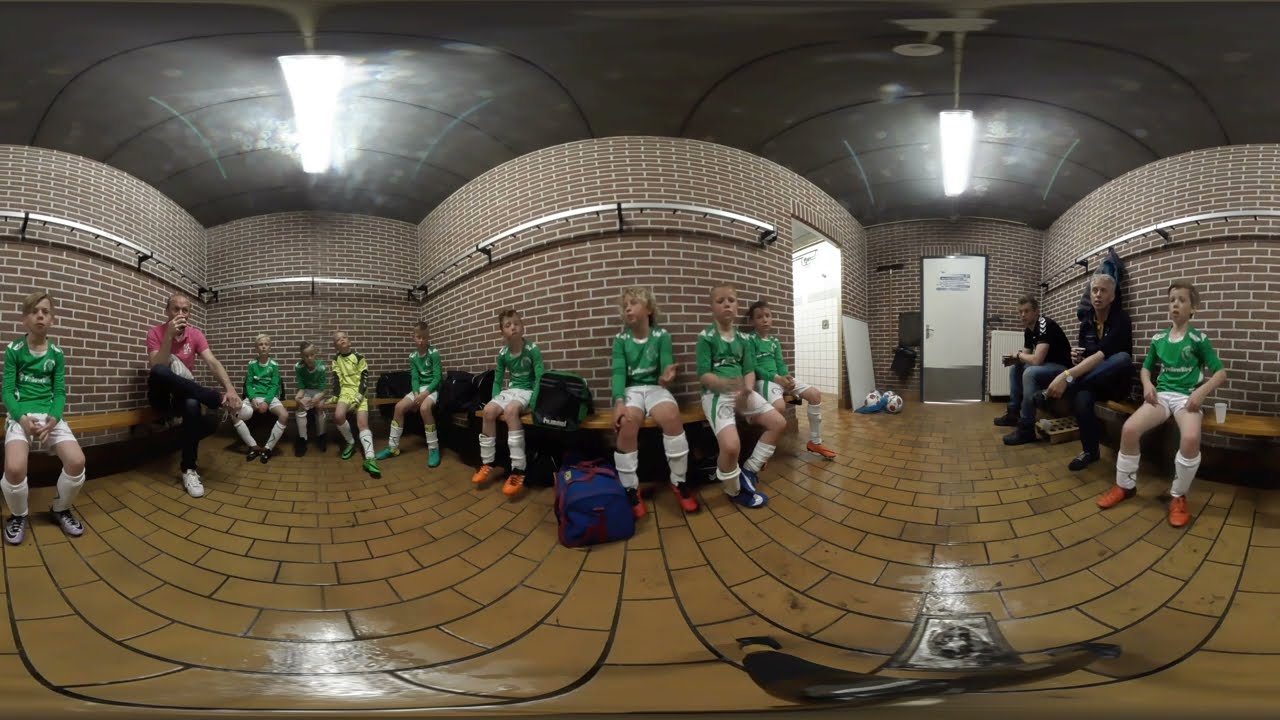In this panoramic image of a middle school locker room, a group of pre-teen children, donned in green jerseys and white shorts with knee-high socks and various colored cleats, sit on benches that line the entire room. This brick-walled area, featuring a shiny brown tiled floor with a visible drain in the foreground on the right, serves as a meeting space for the team before or after a game. The room is illuminated by fluorescent lights on the ceiling, which reflect off the glossy floor. On the left side, we spot two coaches, one in a pink shirt, and another coach accompanied by another man on the right side. In the background, beyond the benches, there's a white-tiled doorway leading to what seems to be a bathroom. Nearby lie scattered soccer balls, and to the far right, we see a white door with a silver kick plate, possibly an exit. Rods above the benches offer a place for hanging jerseys or clothes.